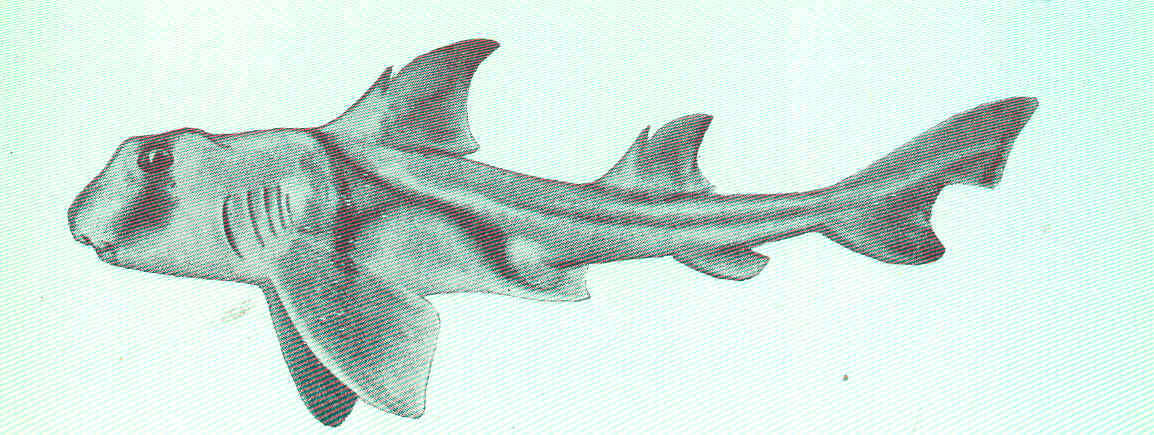The image presents a highly detailed, vintage-style drawing or painting of an unusual, prehistoric-looking shark, centered on a light blue background, possibly from an old textbook or magazine. This grainy, grainy illustration vividly depicts the shark facing left with its tail to the right. The shark sports large, round eyes and features five distinct gill slits on the sides of its flattened head, leading to the assumption it may be a flathead shark. The body is long, sleek, and muscular, showcasing intricate shading in black, gray, and greenish tones.

The front of the shark's body has prominent, wide fins near its mouth, both bottom fins characterized by their notable size. The back reveals two dorsal fins, each tipped with a distinct spike. The triangular tail is unique, marked by a noticeable half-circle notch on the bottom half. The image excludes any text and focuses entirely on the shark, portrayed with enough clarity to see the vertical black lines running along its body and chin, adding to its ancient, almost mythical appearance. This detailed illustration, rich in shades of black, gray, silver, and green, highlights the creature's anatomy in a precise, almost schematic manner, making it suitable for artistic or educational purposes, such as in an art museum or marine biology class.